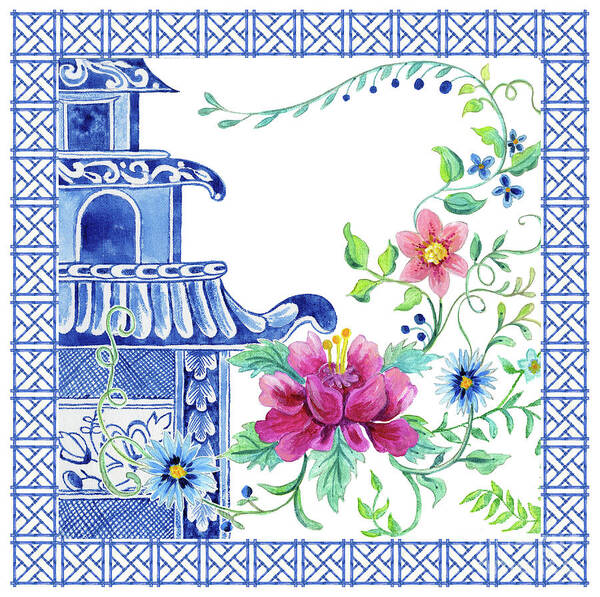This is a detailed and vibrant illustration, likely created with colored pencils, featuring an intricate design that might be suitable for a ceramic tile or a decorative card. The border of the illustration is a repeated blue and white hatch pattern, resembling woven squares, which frames the entire piece. Dominating the left side of the image is an ornate blue and white structure reminiscent of an Asian pagoda or tower. This building shows three levels, each adorned with white flowers, ornate panels, shingles on the roof, and two visible doorways, giving it a detailed and traditional appearance.

On the right side and extending towards the top of the illustration is a lush array of swirling flowers and vines. This floral arrangement includes leaves and foliage in varied hues of dark and light green, interspersed with an assortment of flowers. The flowers range in color from pink and hot pink (with a large rose), to various shades of blue, including cornflowers and other small blue blossoms. There are also elements that resemble blueberries among the vines, adding to the rich botanical tapestry. The combination of the detailed pagoda and the swirling, colorful flowers makes this a captivating and harmonious illustration, showcasing a blend of architectural detail and natural beauty.